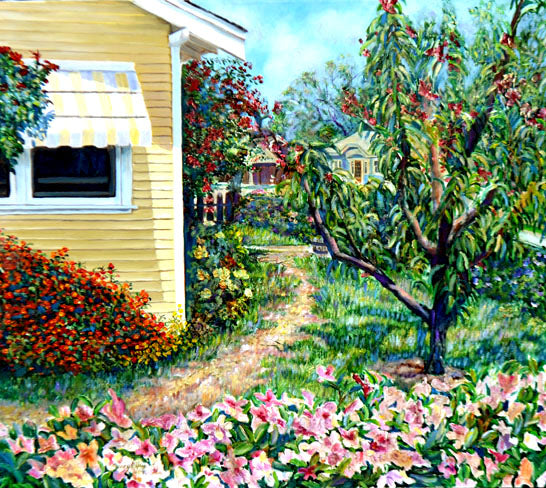This painting vividly depicts a serene residential scene under a clear blue sky with scattered white clouds. The focal point is a charming yellow house with white trim and a yellow-and-white striped awning over a white-framed window. A white pipe runs down the side of the house, and there are two visible windows, with the right one being more prominent. Surrounding the house, the garden is rich with vibrant colors: large bushes adorned with orange, yellow, and red flowers, and an array of pink flowers with green stems spanning the bottom edge of the image. To the right, a wide, branched tree, possibly a cherry tree, flourishes with green leaves and clusters of red flowers. A pathway meanders along the side of the house through a grassy area, creating a picturesque setting. In the distance, additional houses are visible, adding depth and authenticity to this peaceful, residential painting.